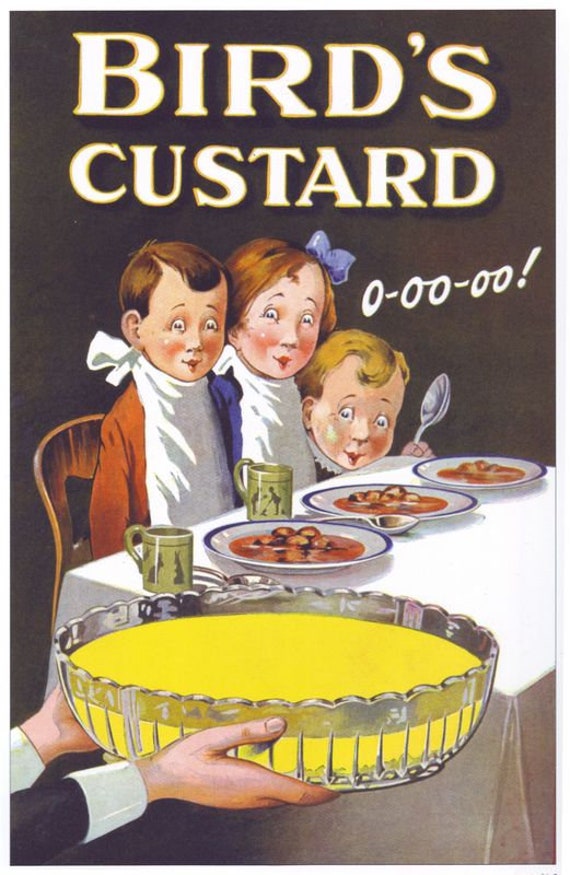The image is a vintage advertisement for Bird's Custard, likely meant for a magazine or newspaper. The ad features a vibrant, cartoony art style. At the top of the image, the words "Bird's Custard" are prominently displayed in large white letters. Below that, three children are seated side by side at a white tablecloth-draped table, ready for dinner. The place settings include white plates with black rims, green mugs, and spoons. The two older children, a boy and a girl, have cloth napkins tied around their necks, while the third child, smaller with blonde curly hair, clutches a spoon in their left hand. All three children are depicted with eager, excited expressions as they gaze at a large metal bowl of yellow custard being presented to them by a person whose black sleeves and white cuffs are the only visible parts. The children's enthrallment with the custard is highlighted by their exclamatory text, "OO-OO-OO!" written in white script next to them.